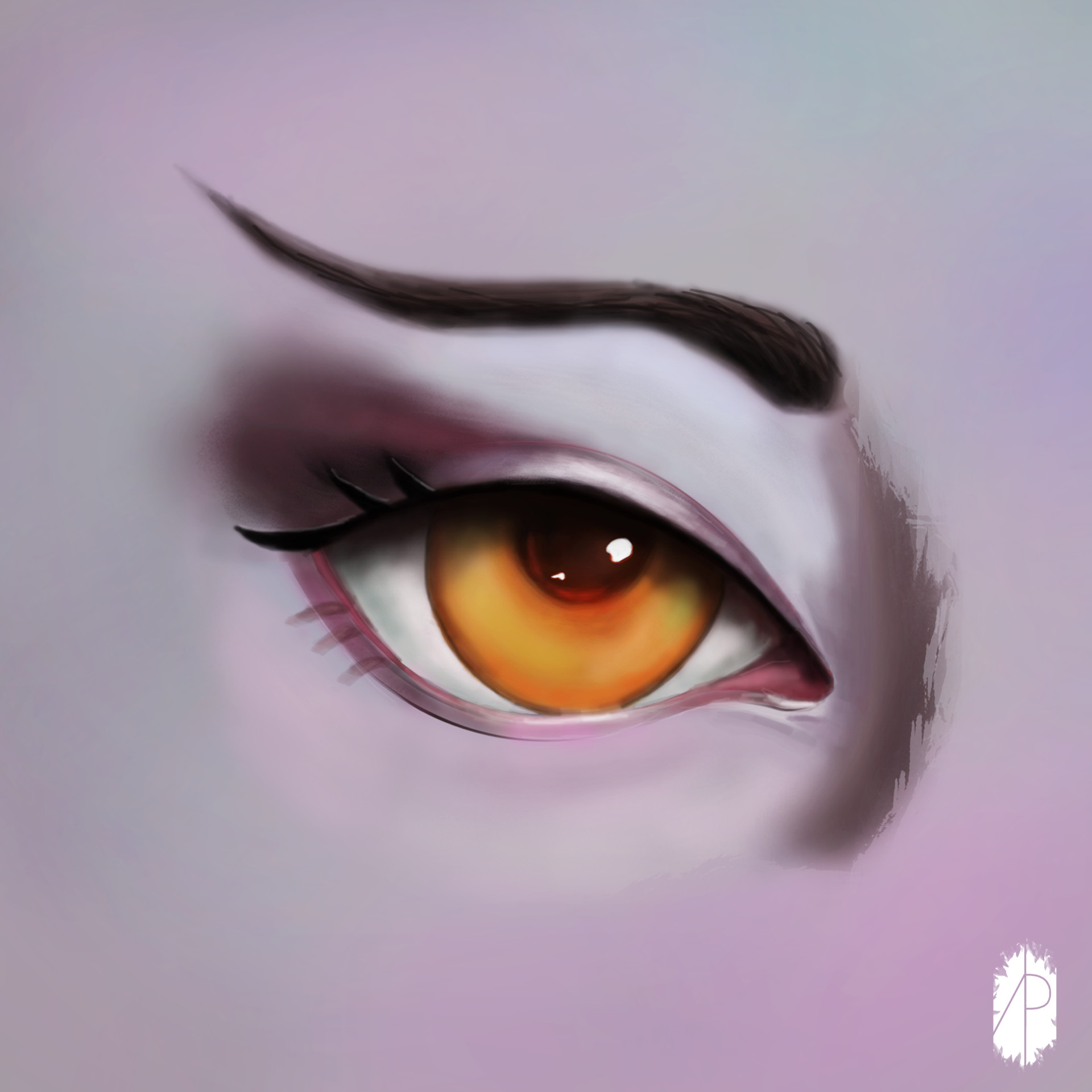The illustration portrays a close-up of a right eye, rendered in vivid, meticulous detail. The skin surrounding the eye is a striking lavender purple, adding a surreal and artistic touch to the image. The inner lid is tinted a reddish purple, and a few sparse eyelashes are visible at the eye's outer corner. A small, dark eyebrow arches above. The artist has skillfully used shading to depict the contours of the face, particularly around the tear duct area and the outer top corner of the eyelid, suggesting the bridge of the nose and possibly eyeshadow. The eye itself features a brownish pupil with two white reflections of light, the larger reflection dominating the smaller one. The iris has a hazel hue, blending brown and green tones. An artist's signature, a stylized conjoined A and P in a feathery white shape, is placed in the bottom right corner of the image, marking the creator's unique touch.